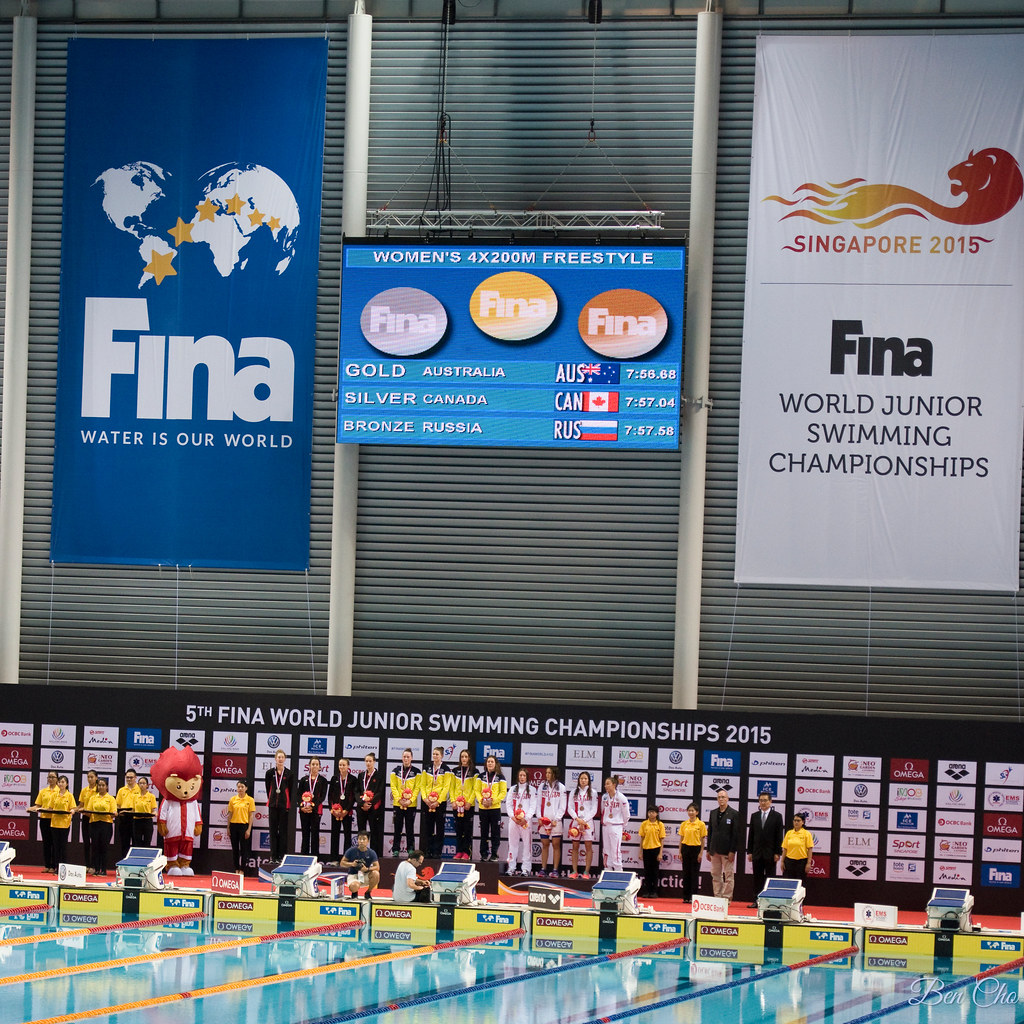The image depicts an awards ceremony at the 5th FINA World Junior Swimming Championships 2015, held in a large indoor swimming arena. The scene captures the winners of the Women's 4x200 meter freestyle event lined up in front of a pool with light blue water, divided into lanes by multi-colored ropes. A prominent display behind them includes various sponsor logos and banners. Central to the image are groups of competitors, with the gold medalists from Australia, the silver medalists from Canada, and the bronze medalists from Russia, identifiable by the medals around their necks. Participants and staff are dressed in a variety of outfits, ranging from black and yellow uniforms to all-white attire and golden shirts. A digital screen above the group displays the event details: "Women's 4x200m Freestyle," with the results showing Australia taking gold with a time of 7:56.68, Canada silver at 7:57.04, and Russia bronze at 7:57.58. Beside the screen, banners read "FINA, Water is Our World" and "Singapore 2015 FINA World Junior Swimming Championships," accompanied by a logo featuring a flaming lion. The scene is further animated by the presence of a mascot in a red costume, adding to the celebratory atmosphere.